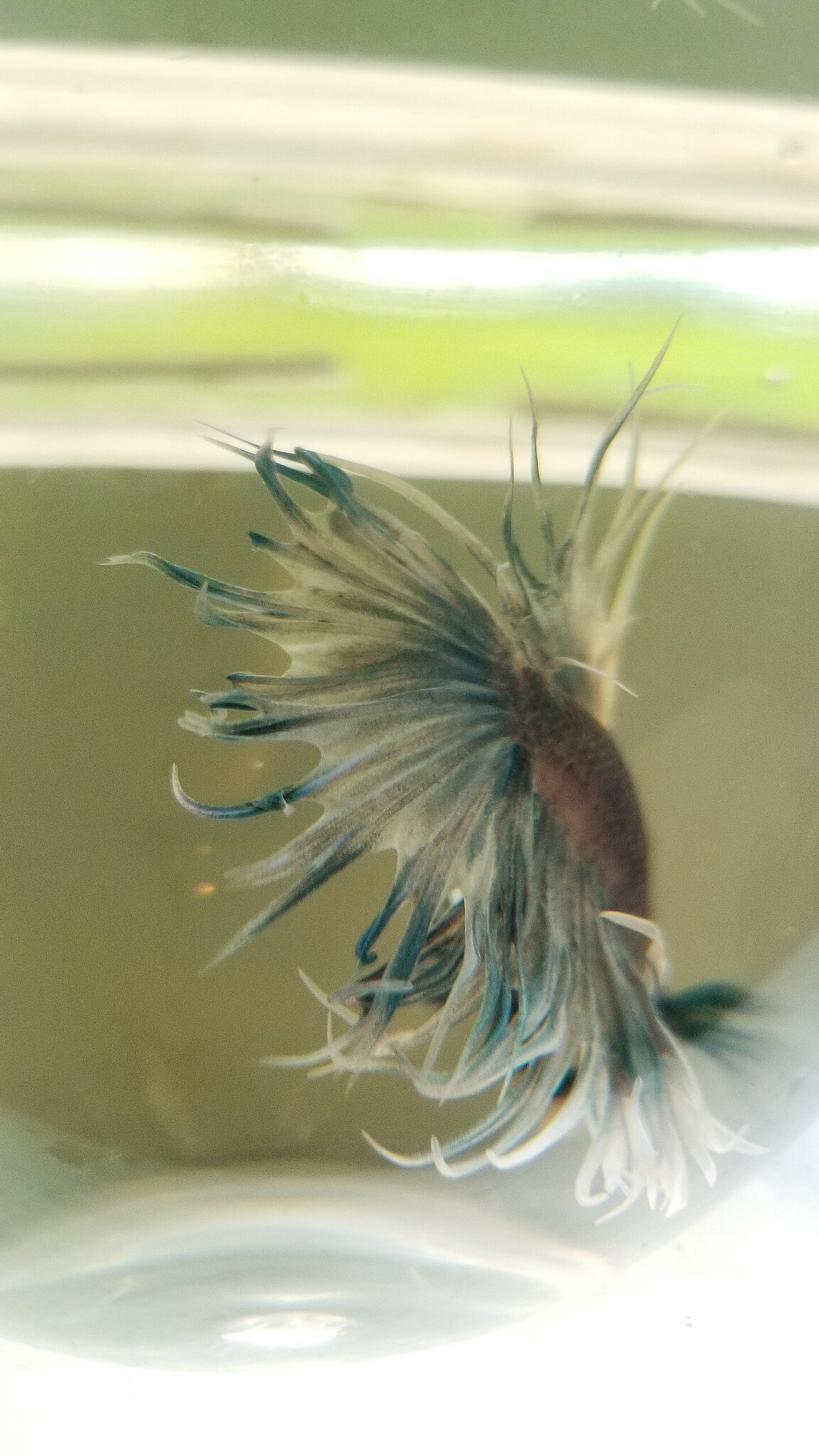In this detailed, outdoor day-time photograph, the setting appears to be a unique and intriguing scene. At the forefront is a curious aquatic creature that resembles a blend between a sea animal and a floral organism. Its body is furry with vibrant green and yellow hair, radiating from a central, face-less core that looks reminiscent of a sunflower. This anomaly is perched on a curved gray surface, transitioning into a light green grassy plot. The fish-like figure, or perhaps a sea creature, has an affinity to a Japanese fighting fish or Siamese fighting fish, boasting colorful purples, whites, and blues, especially noticeable on its long, tentacle-like fins which are somewhat fluffy, akin to jellyfish limbs.

In the mid-ground, slightly out of focus, there is a light green lawn alongside two dark, gray rectangular shapes. These give way to a body of water, reflective in shades of gray and white. Beyond the water, there's a band of sand followed by another patch of green grass, all adding to the layered depth of the background. The photograph is free of text, allowing the viewer to immerse fully in the enigmatic beauty of the scene, which is both captivating and puzzling, revealing an enthralling blend of terrestrial and aquatic elements.